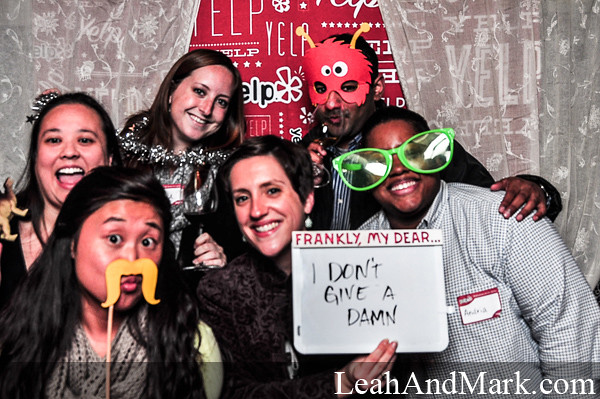This is a vibrant color photograph in landscape orientation capturing six people in various playful costumes, evidently celebrating. They are all smiling and looking up at the viewer, with their arms around each other. Centered in the image, a person holds a white sign with red and black letters that reads "Frankly, my dear, I don't give a damn." This person, an African-American wearing oversized bright green glasses and a white shirt with black and blue checkered stripes and a name tag on their left chest, stands out with a sign prominently displayed.

To the left of this person, another individual in a white shirt with black stripes and a name tag is holding up a red mask with protruding ears, resembling a bug. Beside them, there's a woman with short black hair in a dark sweater, smiling brightly. Another woman with long black hair, wearing a white blouse, is holding a stick with a yellow fake mustache next to her nose. 

The background features a pale gray curtain and a red wall sign adorned with the Yelp logo, providing a festive atmosphere. Text at the bottom right corner reveals the photography credit, "Leahandmark.com." This lively scene showcases the diverse and joyful spirit of the group, underscored by the playful elements of their costumes.